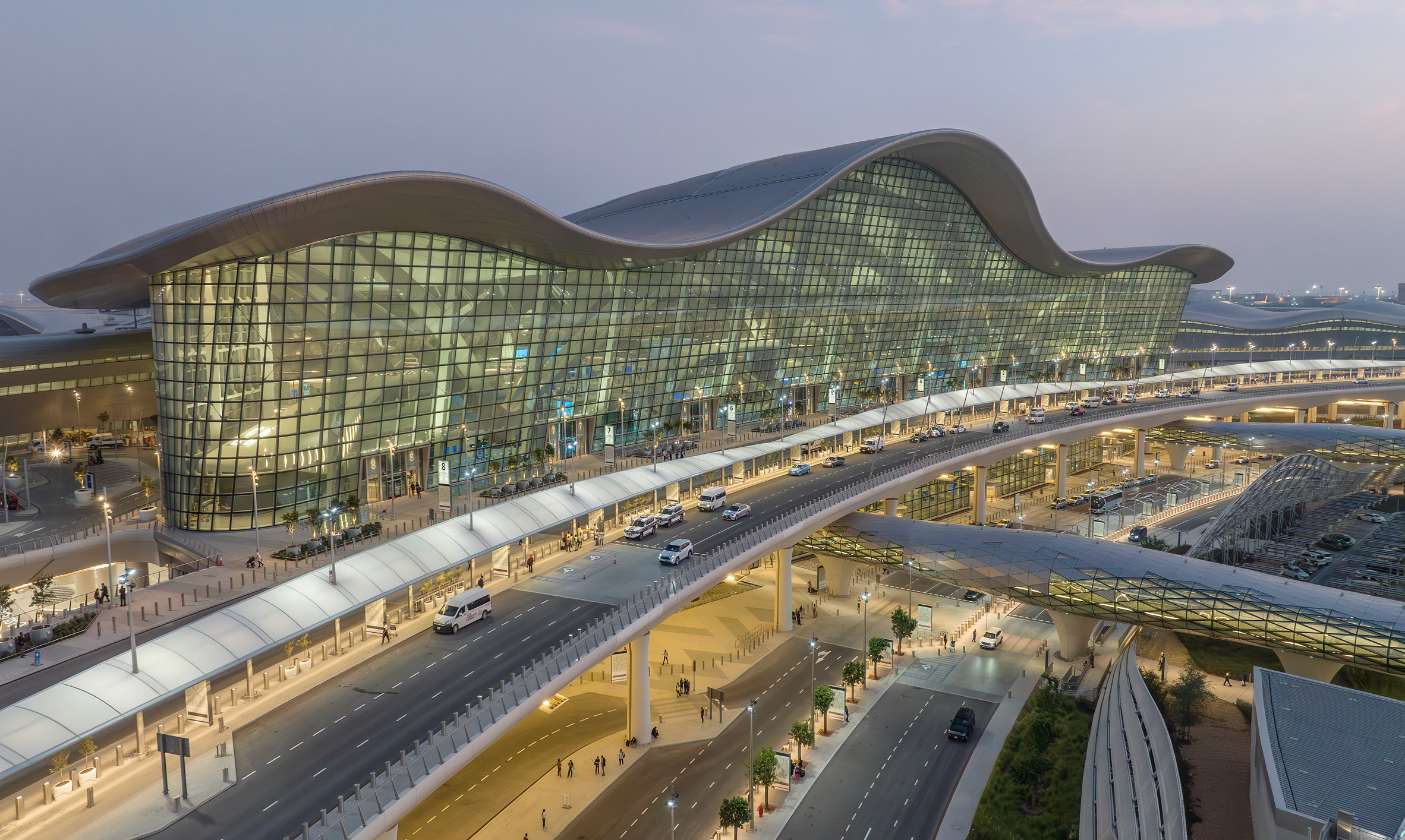This aerial photograph, likely taken by a drone, captures a twilight view of an airport terminal. The central focus is a massive, glass-covered structure with a distinctive wavy, silver-colored roof. The facade is composed of numerous square glass panels, with larger panels on the ground floor and smaller ones higher up. The terminal's elegant architecture echoes the grandeur of a high-end hotel or stadium. Multiple levels of access roads snake around the building, allowing cars, vans, and buses to drive up or park. Pedestrian bridges and walkways connect these different levels, bustling with activity. Below the main building, a garage-like structure accommodates further vehicular movement and parking. The image radiates a soft, greenish tint from the illuminated glass, enhancing the scene's twilight ambiance. In the distance, similar curved-roof buildings and highways adorned with moving vehicles add depth to the composition. The sky's bluish-gray hue and the professional quality of the photograph accentuate the overall ethereal and intricate nature of the terminal's design.